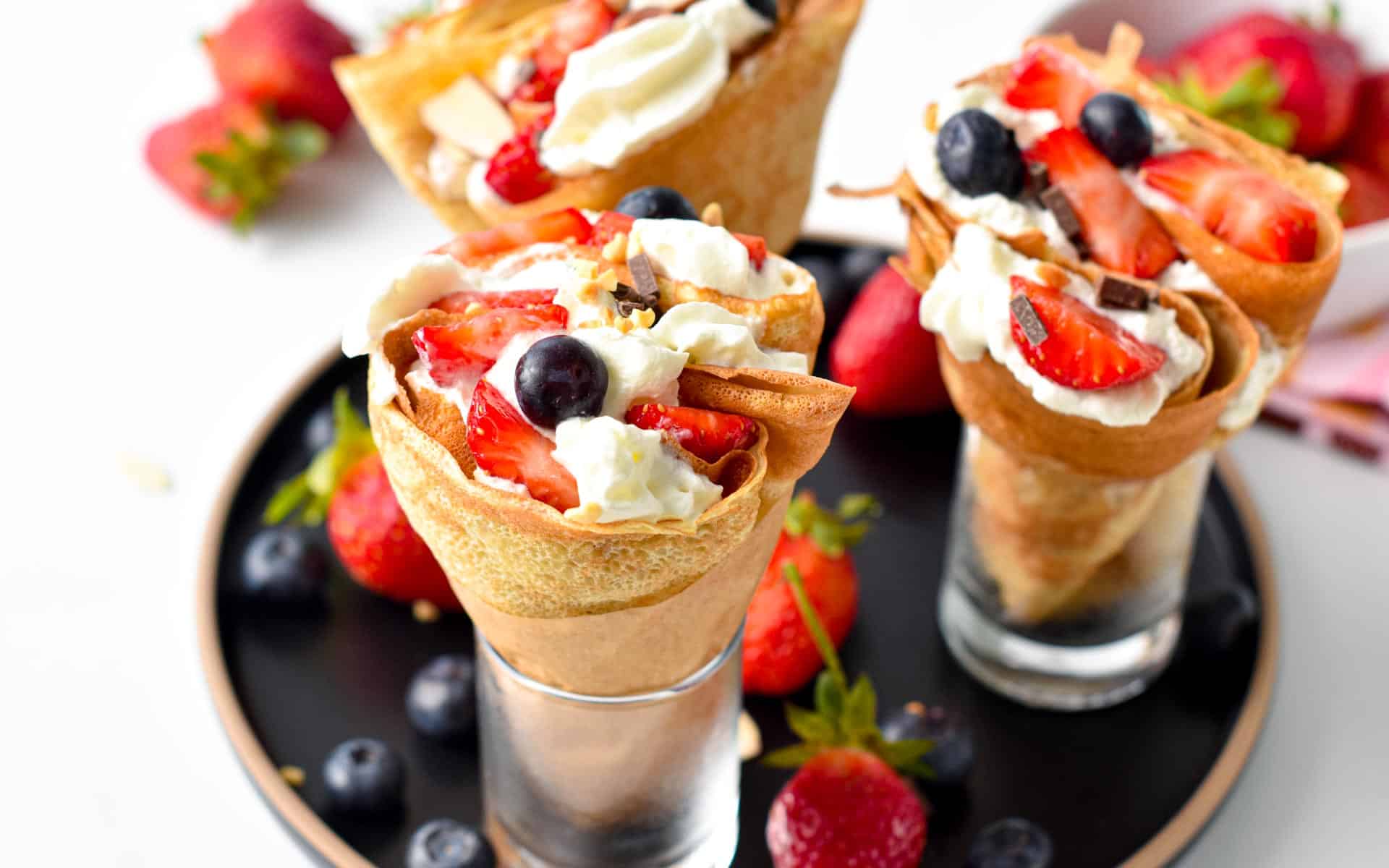An overhead shot showcases three crepe cones filled with luscious whipped cream, sliced strawberries, and blueberries, garnished with delicate chocolate shavings. Each cone, expertly rolled into a conical shape, is nestled in a small, clear glass serveware placed on a black tray with a bronze border. Scattered around the tray are loose strawberries and blueberries, adding a vibrant burst of color against the dark background. The tray rests on a white table. Out of focus in the background, a bowl of fresh strawberries can be seen on the right, while a couple of strawberries lay on the left. The composition, with its rich array of reds, blues, tans, and blacks, evokes a sense of delectable indulgence.